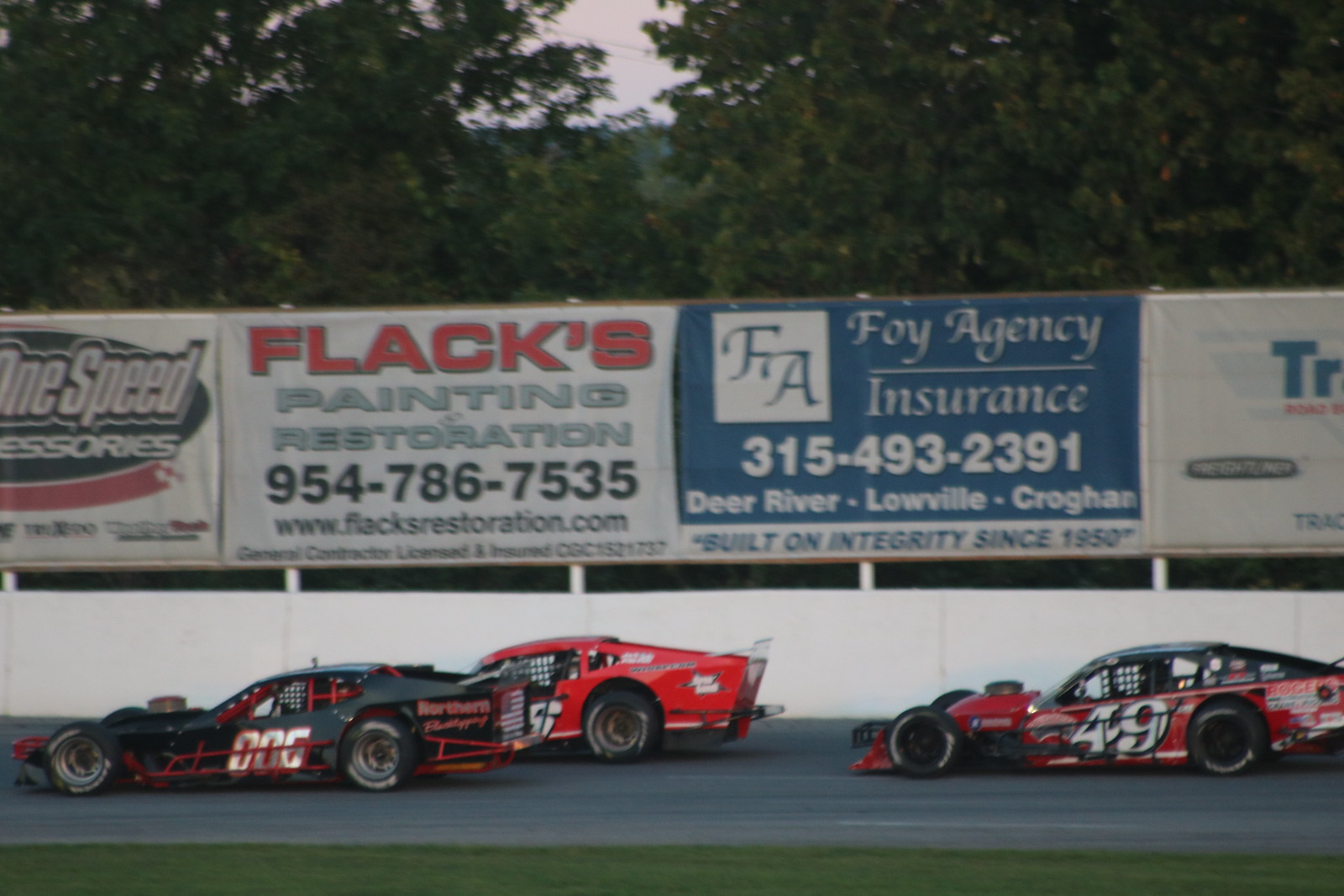This color photograph captures an active NASCAR-style race at a racetrack, vividly depicting the dynamic atmosphere of the event. In the foreground, there is a patch of grass leading to the grayish-black asphalt of the speedway. Three race cars dominate this scene, racing side-by-side. The leading car, numbered 006, is predominantly black with red and silver lettering. Slightly behind it is a red car, bearing the number 6. Trailing these two is another car, strikingly red with a black hood, marked by the number 49 in white.

Behind the speeding cars lies a white wall, capped with a series of billboards displaying various advertisements. The advertisements include "Flax Painting Restoration" with contact information listed as 954-786-7535 and a website, www.flaxrestoration.com, followed by a billboard for "FOI Insurance Agency," which reads "built on integrity since 1950," and lists locations in Deer River, Lowville, and Krogan, along with a contact number 315-493-2391.

Further back in the image, beyond the advertisements, stands a row of trees, adding a contrast of green foliage against the industrial backdrop of the racetrack.